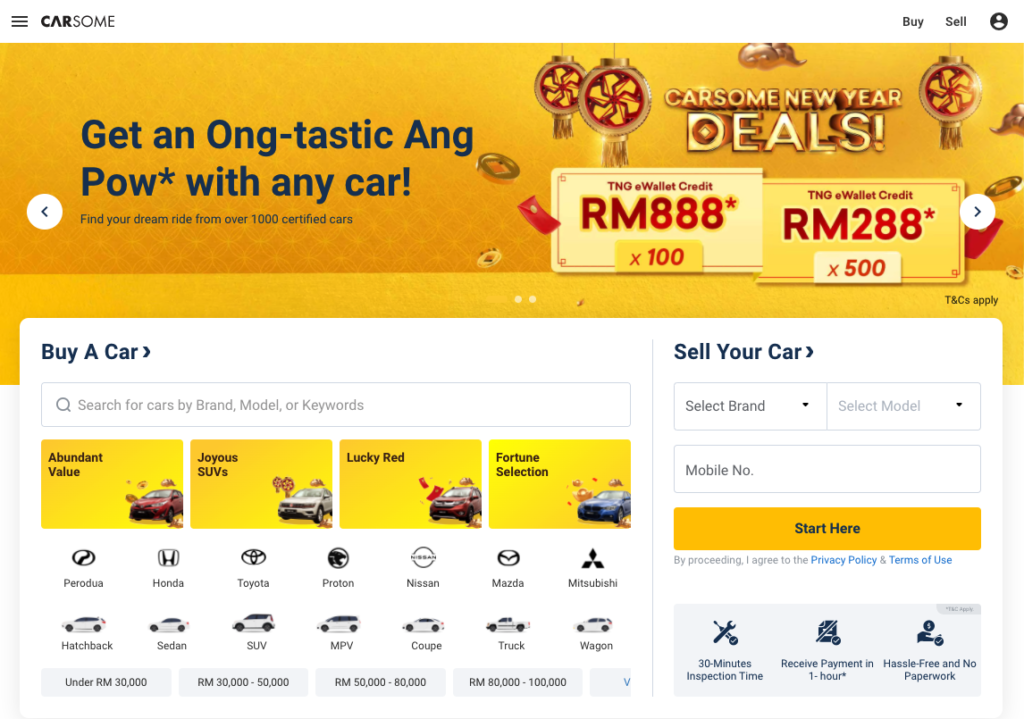Certainly! Here's a cleaned-up and detailed caption for the image described:

---

This is a screenshot of the CarSum app interface. At the top left, there's a menu icon, followed by the "CarSum" logo. To the right within the menu bar, there are three options: "Buy," "Sell," and a profile picture icon, all set against a white background. Below this is an eye-catching orange header, featuring the text "Get an Ong-tastic Ang Pal with any car" and "Find your dream ride from over a thousand certified cars," written in dark blue.

Navigation arrows to the left and right indicate that you can scroll through the header images. On the right-hand side, there are decorative decals resembling license plates. These display "TNGE Wallet Credit RM888" and "RM288" with a star symbol next to the numbers. Below these, in bright red text on a yellowish background, it says "x100."

Above the two license plate graphics, the promotional text "CarSum New Year Deals" is prominently displayed. Below this, a white box contains the option to "Buy a Car." Underneath is a search bar allowing users to search for cars by brand, model, or keywords. Further down, there are selections for different car brands with corresponding buttons.

On the right side, there is a section for selling cars. This includes fields to select the car brand and model, as well as a space to enter a mobile number, followed by a "Start Here" button. Additional information about selling a car is displayed below this section.

---

This detailed caption aims to provide comprehensive information about the various elements and features presented in the CarSum app interface.